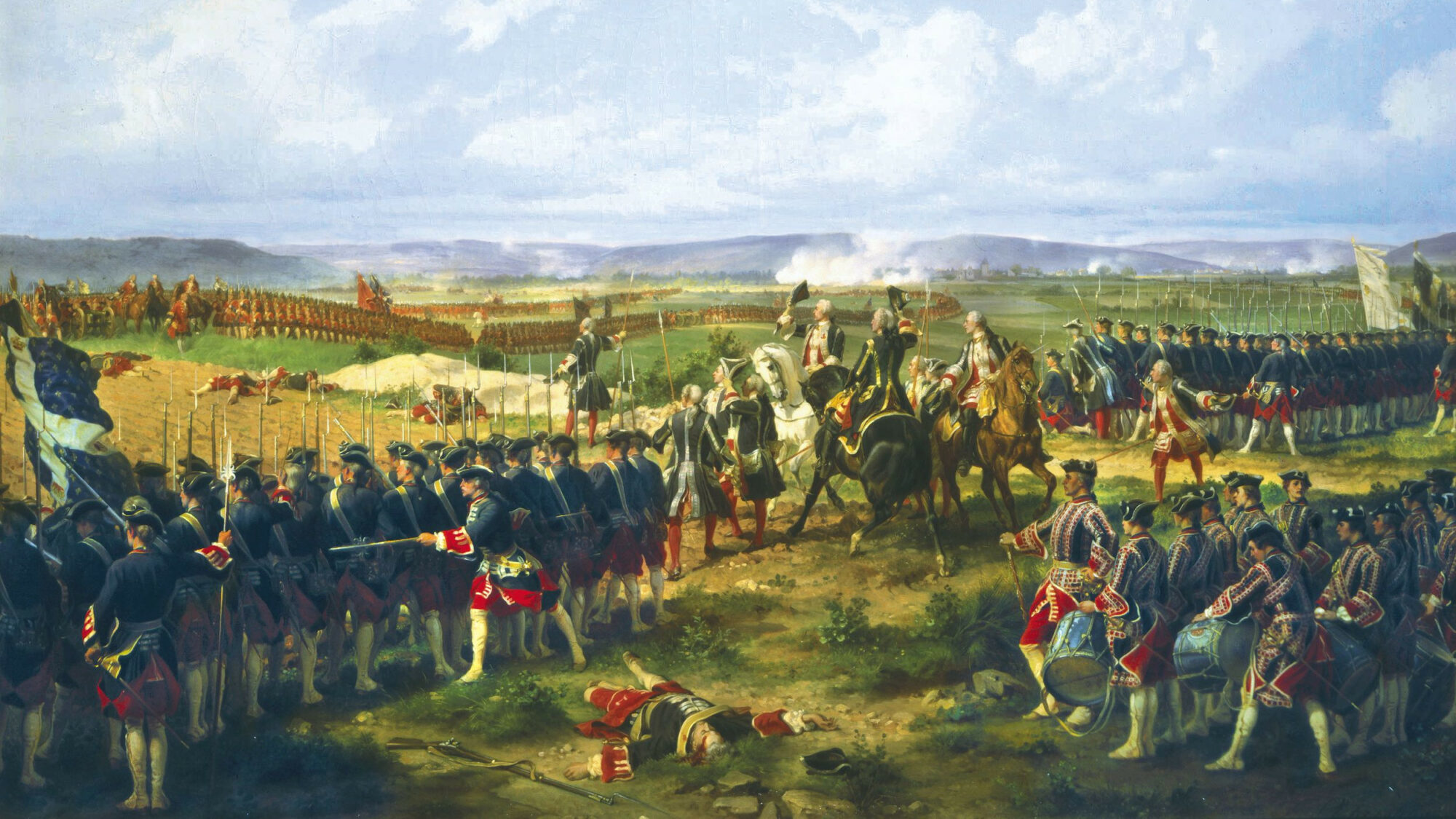This painting captures a detailed scene of a daytime battle, evocative of either the Revolutionary War or the Civil War, staged on a hilly open field under a sky filled with wispy white clouds. To the left and right, lines of soldiers in dark blue and red uniforms, respectively, stand in formation. The men in blue are closest to the viewer, equipped with old-fashioned rifles, muskets with bayonets, and some wearing black hats. Musicians playing drums are interspersed among them.

In the center, three commanders on horseback—a white, black, and brown horse—observe intently, having removed their hats. Their uniforms feature intricate details, including golden accents and knee-high white boots. Their distinctive white, braided, ponytail wigs suggest a historical European connection, supporting the notion of a British or Colonial army.

Further back, the opposing line of soldiers, clad in reddish uniforms, stands visible, with large, billowing white smoke rising from several areas—possibly indicating recently fired volleys or campfires. A range of hills and distant blue mountains complete the landscape, accentuating the tension and anticipation of the impending battle.